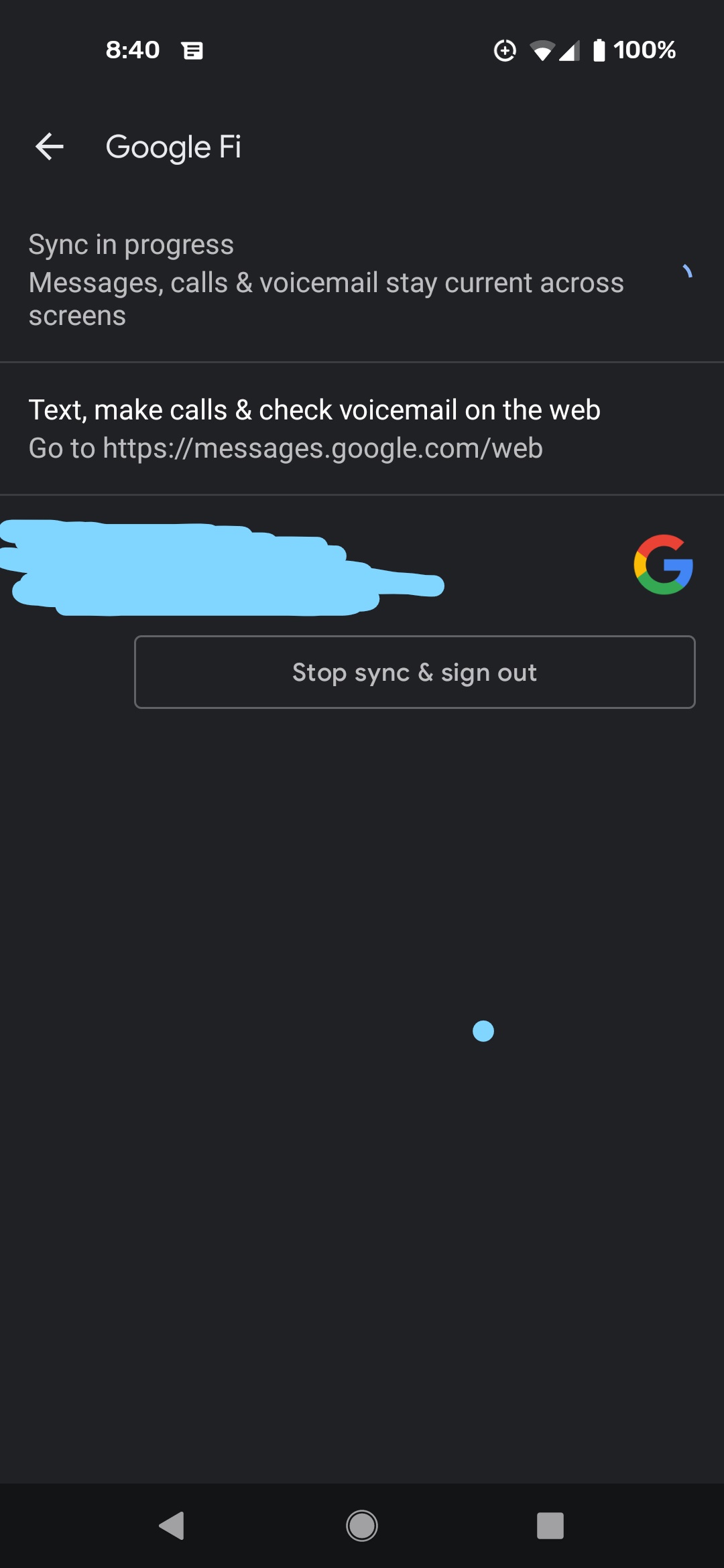The image features a dark gray background with various interface elements. In the upper left corner, it displays "8:40" in white, indicating the time. To the right of the timestamp, there's a white messaging icon, followed by a circular icon with a slit at the top, containing a white plus sign at its center. Continuing to the right, there's a Wi-Fi signal icon, a data bar symbol, and a fully colored white battery icon indicating 100% charge, accompanied by the text "100%" in white.

Below this line, there's a left-pointing arrow suggesting navigation to a previous menu, next to which it reads "Google Fi" in white text. Beneath that, in medium gray, it states "Sync in progress," followed by the message "Messages, calls, and voicemail stay current across screens." This message is separated by a thin, light gray divider from the next section, which reads "Text, make calls and check voicemail on the web" in white text. Below this, in light gray, is a URL: "https://messages.google.com/web."

Further down, there's an area obscured by light blue scribbles, likely for privacy reasons. To the right of this blocked-out section is the Google logo, a stylized "G" with a red top, yellow left side, green bottom, and blue tail. Below the logo, a long rectangle outlined in light gray contains the text "Stop sync and sign out" in white, placed in the center of the rectangle.